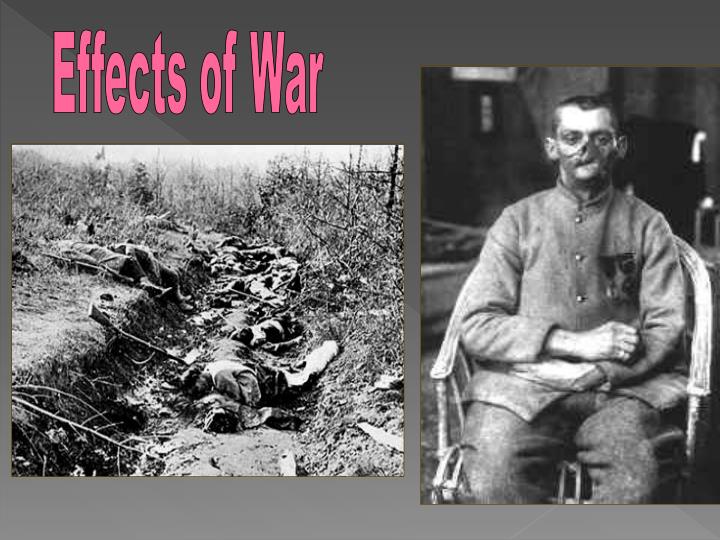On a gradient gray background transitioning from darker at the top right to lighter at the bottom left, large pink text in block letters reads "Effects of War." Below, two black and white photographs are separated by a faint diagonal line. The left photo depicts a somber scene: a trench filled with corpses, some lying amidst sparse, lifeless trees and muddy grass, likely signifying a fall or winter setting. The right photo centers on a man in a wicker chair, draped in an old-fashioned war uniform. His face is heavily disfigured and covered, presumably from wartime injuries, and one of his arms appears misshapen or injured. His posture is upright with arms folded over his abdomen, looking directly at the camera, solemn and reflective.